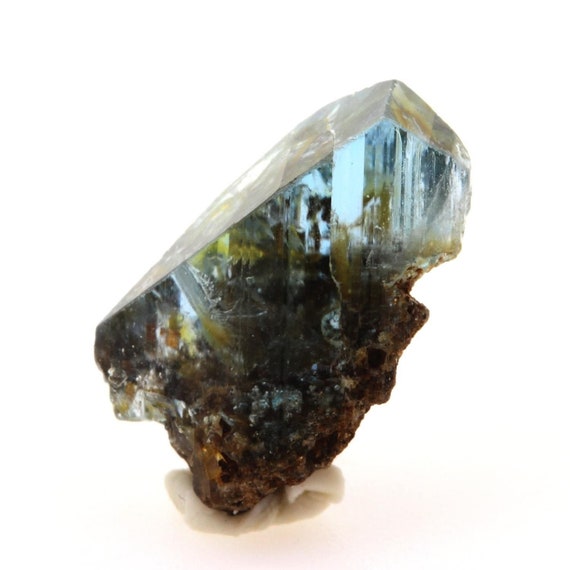The image depicts a crystalline mineral perched atop what appears to be a piece of chewed white gum. The mineral, which is semi-transparent on the upper portion, features a flat surface and triangular tip on the upper left, while the upper right is comparatively shorter. The top of the mineral is almost see-through with faint lines and yellow hues. In contrast, the lower half of the mineral is brown, rough, and more rock-like in texture. The gum underneath serves as an improvised platform, creating a stark visual juxtaposition between the crystalline upper part and the earthy, opaque lower section.